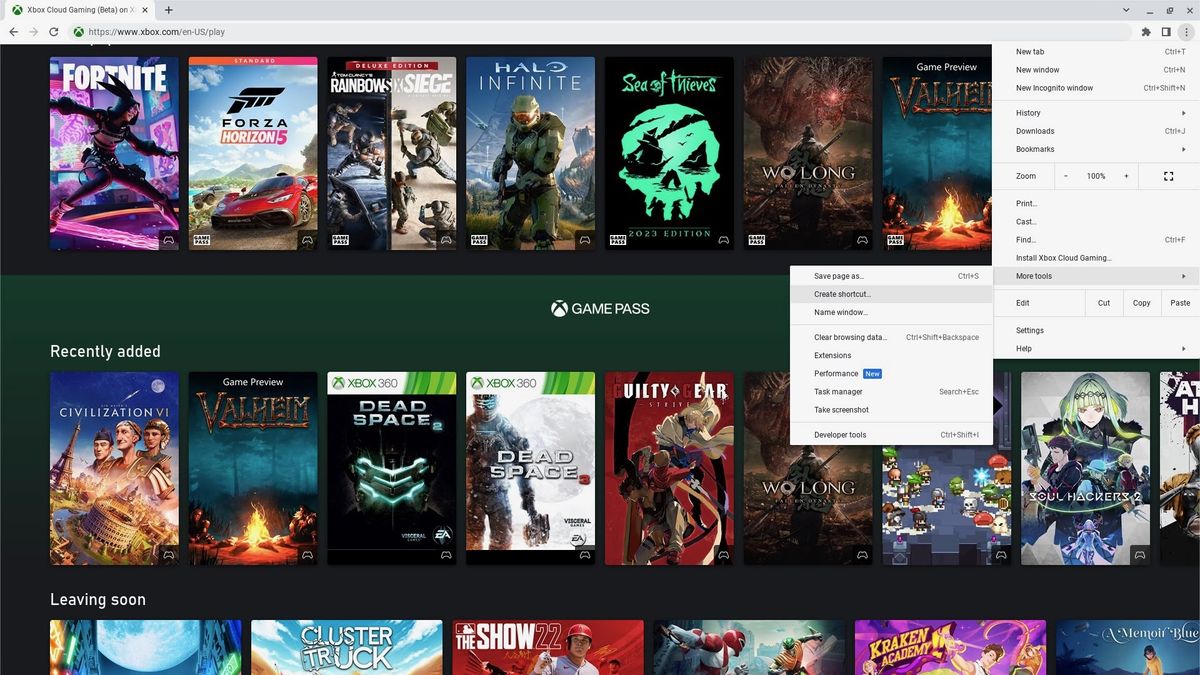The screenshot depicts the Xbox Cloud Gaming (Beta) website, specifically located at xbox.com/en-us/play. The web browser displays a single tab, with a black background on the top strip. The content of the tab prominently features popular game titles such as Fortnite, Forza Horizon 5, Rainbow Six Siege, Halo Infinite, Sea of Thieves, Wo Long, and Valheim, although the latter part of the list is cut off.

In the upper right corner, a drop-down menu is open, revealing various browser options. The menu includes the following items: New tab, New window, New incognito window, History, Downloads, Bookmarks, Zoom (100%), Print, Cast, Find, Install Xbox Cloud Gaming, More tools, Edit, Settings, and Help. The 'More tools' submenu is expanded, showing further options like Save page as, Create shortcut, Name, Window, Clear browser data, Extensions, Performance (New), Task manager, Take screenshot, and Developer tools.

Overlaying this menu is the central content of the webpage, which features the iconic Xbox Game Pass branding.